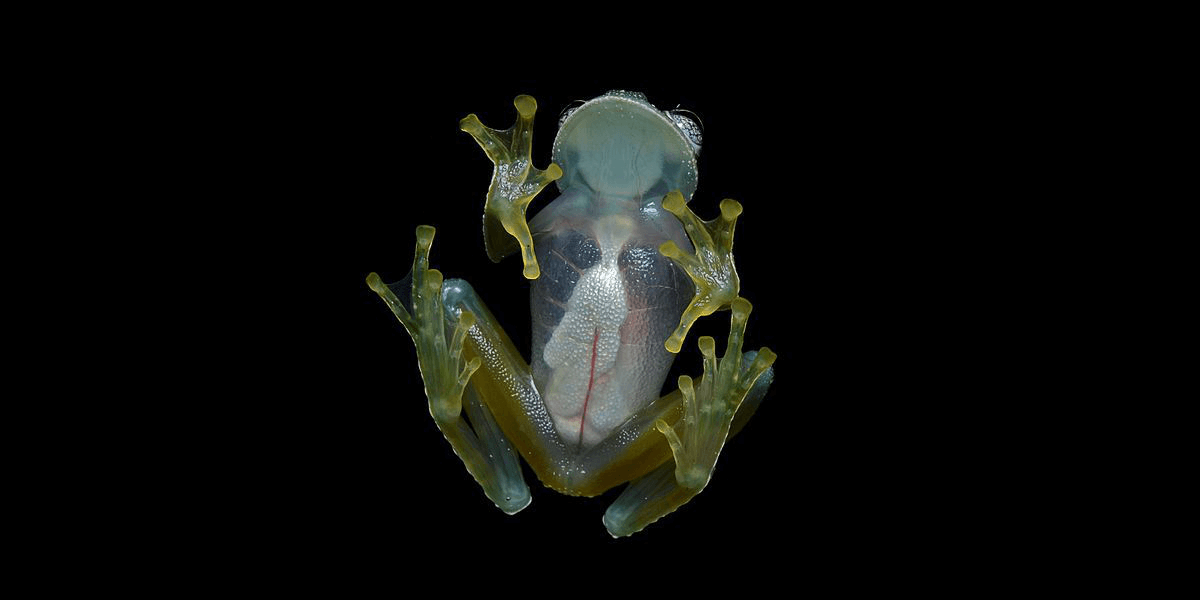This detailed photograph captures the unique underside of a green frog set against a black background. The image reveals the frog's translucent body, allowing a glimpse into its internal structure. Visible under the frog's pale bluish head are its silver-colored intestines and a prominent red blood vessel running from its chest to its pelvic area. The frog's torso is almost colorless, offering a clear view of its internal organs, while its legs and arms showcase a translucent green hue. Each digit is equipped with what appear to be suction pads. The frog is lying on a see-through glass surface, giving a relaxed pose, with one eye just visible. This remarkable view highlights the intricate details of the frog's anatomy, showing the beauty of its webbed feet and the pale green under its tongue.